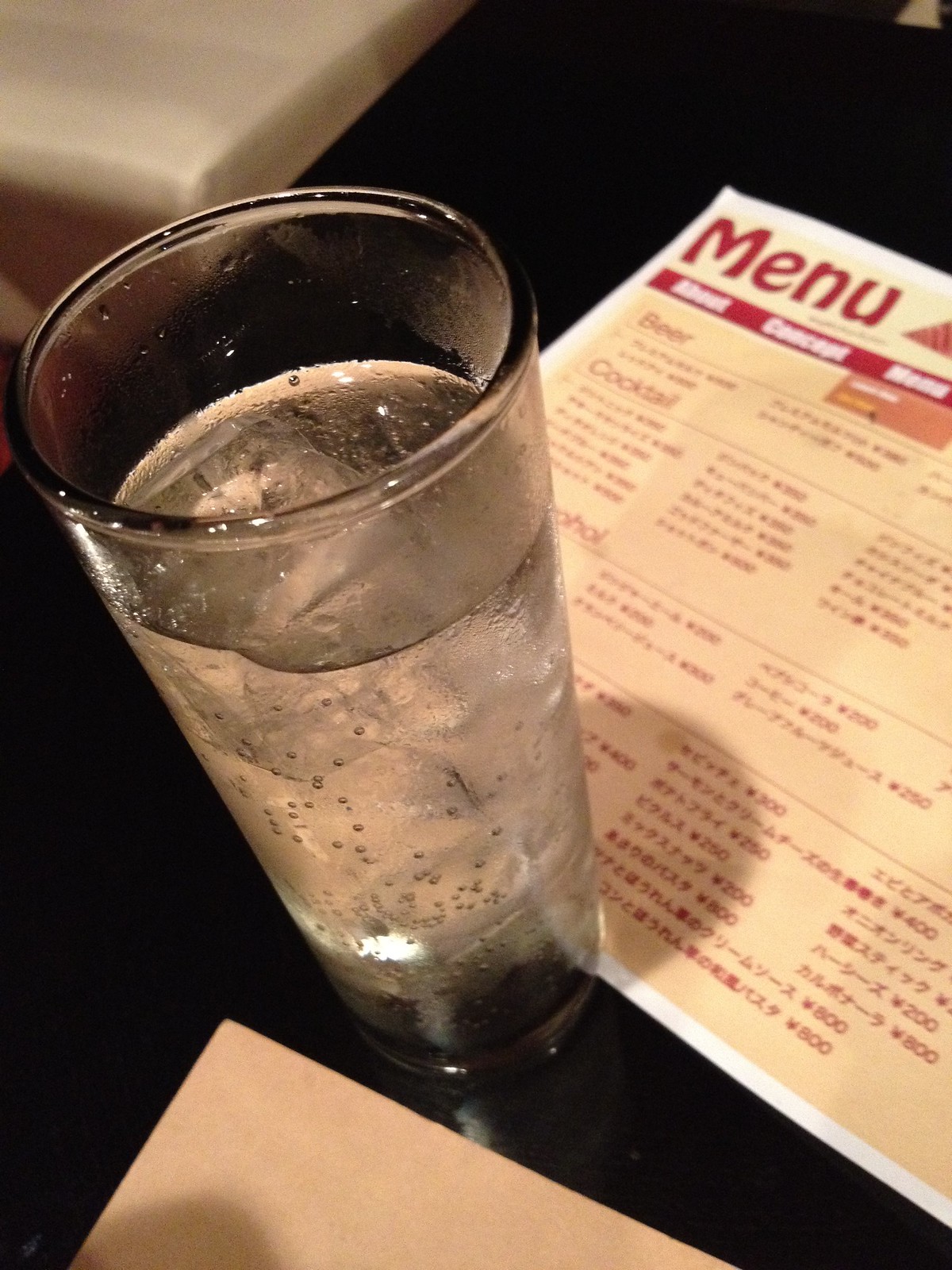This detailed photograph captures a clear glass, filled approximately 80% with sparkling water and ice cubes, placed on a black table. The glass, which is smooth and cylindrical with slight inward tapering near the base, stands prominently in focus. Beside the glass sits a beige-colored menu adorned with red and occasional white writing. The word "menu" is distinctly featured at the top in bold red letters, while the menu items are written in Chinese or Japanese, with English text listing "beer," "cocktail," and "alcohol." In the bottom left of the image, another sheet of similar off-white color lies blank. The background reveals a glossy, flat black table and glimpses of a table draped in a white tablecloth, all suggesting the setting is an Asian restaurant.